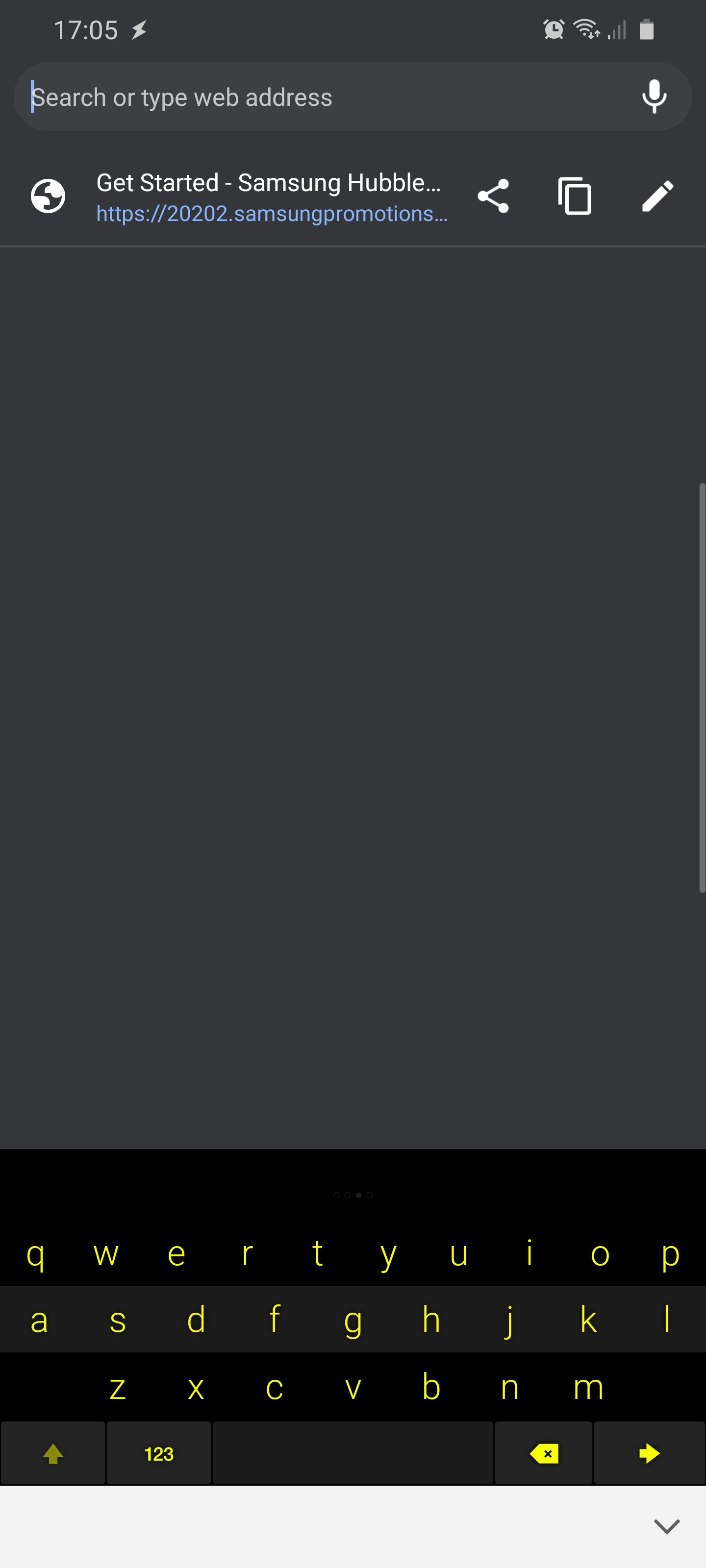The image displays a screenshot from a cell phone.

In the upper left-hand corner, "1705" is shown in gray text accompanied by a lightning bolt icon. On the upper right-hand corner, there are several status icons: an alarm clock, a Wi-Fi signal, a cellular signal with one bar highlighted, and a battery indicator showing approximately 80-90% charge.

Just below these icons is a search field labeled "Search or type web address," with a blue vertical line on the left side of the box and a microphone icon on the right. Below this, there's a circular S-shaped logo accompanied by the text "Let's get started, Samsung Hubble" in white, and a hyperlink in blue to "Samsung Promotions" beneath it.

Three icons are situated below this text: a share icon, a copy icon, and a pencil icon, all separated by a thin gray line. Toward the bottom of the screen, a standard keyboard is visible, featuring yellow font on a dark black and gray background. The keyboard includes special buttons for switching to numbers, a delete arrow, and a forward arrow.